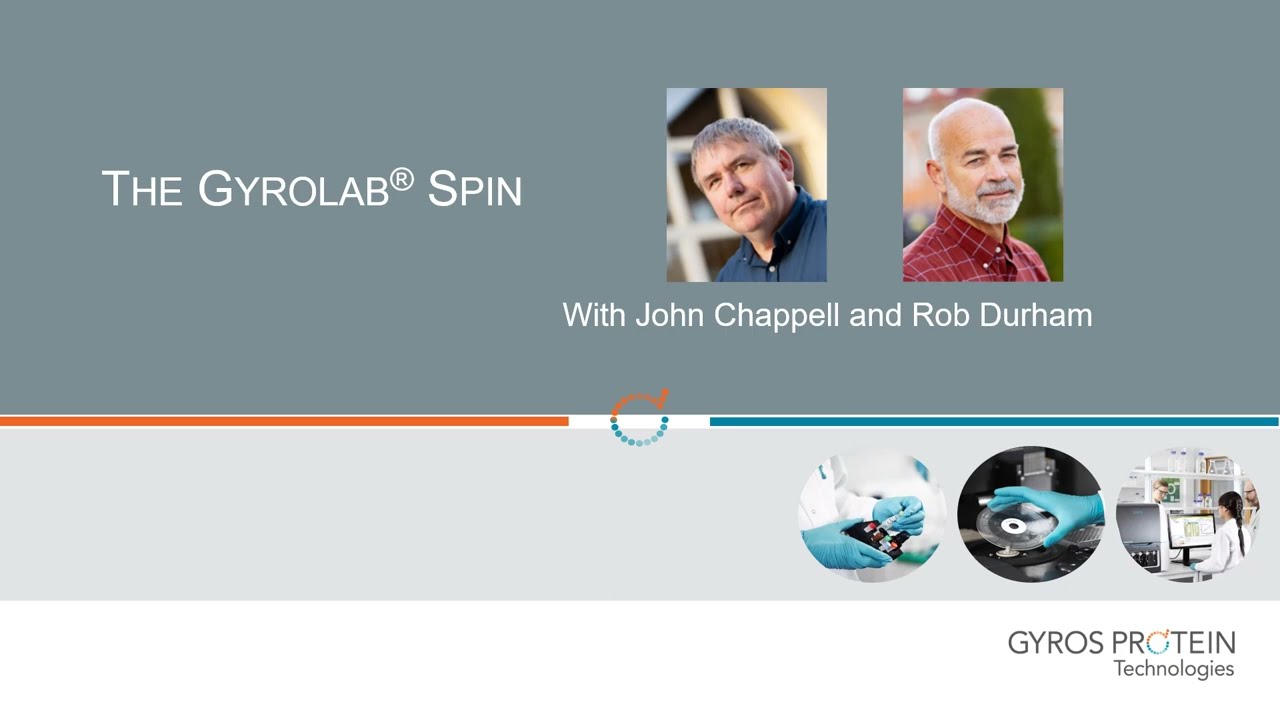The image serves as the title slide for a PowerPoint presentation introducing the Jarrow Lab Spin product. The text at the top-left identifies the product name, "Jarrow Lab Spin," accompanied by a registered trademark symbol. This central text sits against a gray background. Surrounding it are two headshot images, one of John Chappell in a blue button-up shirt with gray hair and a serious expression, and another of Rob Durham in a red and white checkered button-up shirt, sporting a white beard and bald head. Their names appear beneath their respective images. At the bottom right of the slide, the logo for Jarrow’s Protein Technologies is displayed. Additionally, this section includes smaller concept images related to the technology—one shows gloved hands interacting with a digital object, another depicts green-gloved hands holding a petri dish, and the last image shows a scientist working at a computer in a lab setting. The entire layout, dominated by the company’s orange and blue colors along with white and black text, suggests a polished and corporate visual style, likely intended for a professional presentation setting.